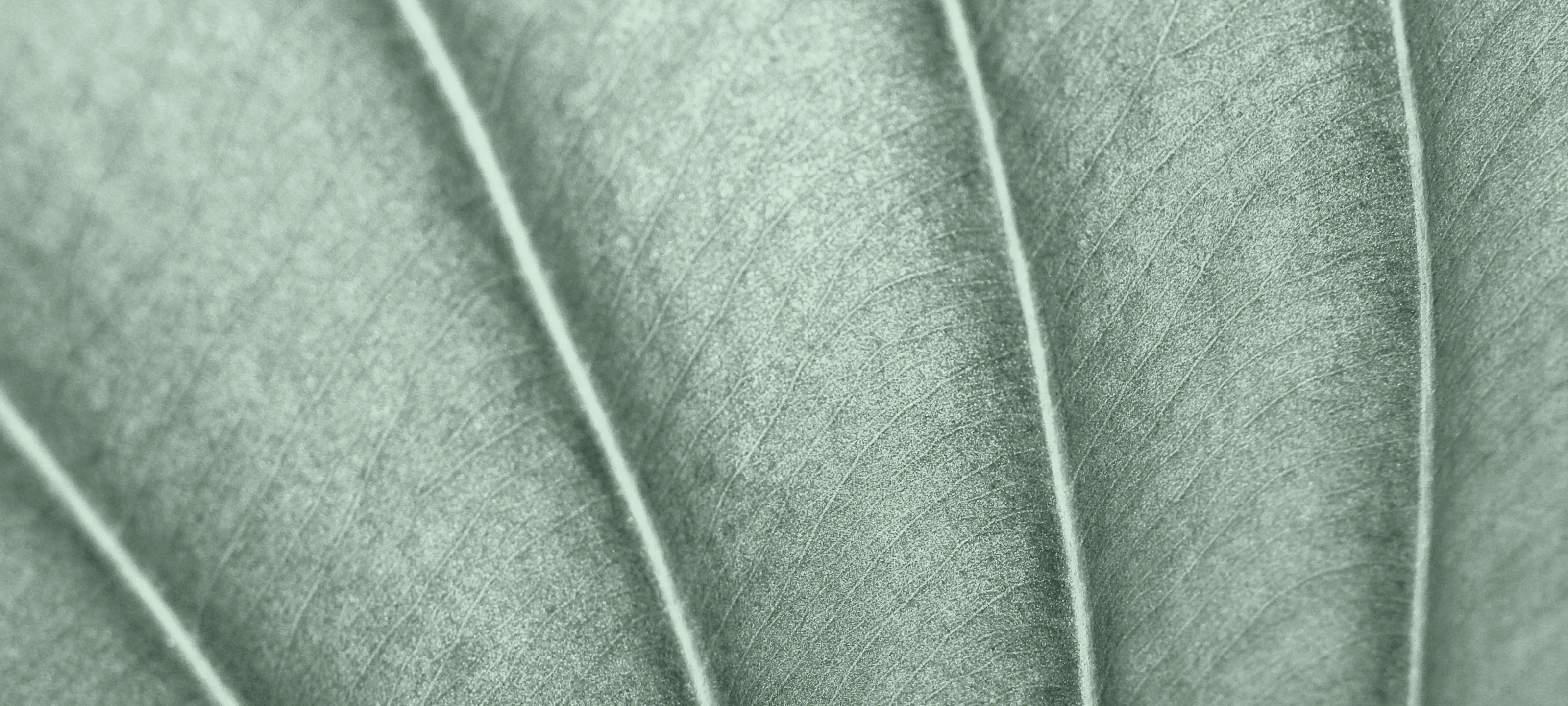The image displays a detailed, close-up view of a leaf, potentially a painting or a highly realistic photograph. The leaf is characterized by light green textures and intersected by white to greenish veins, creating a network reminiscent of the intricate patterns found in plant leaves. The composition is divided into five vertical rectangular sections, although the far-left section is only partially visible and the far-right section is about a quarter of one of the central sections' width. The leaf's texture exhibits horizontal lines, and it features noticeable white patches and green pores. The interplay of these elements, coupled with the leaf's green and grayish tones, raises questions about whether the image is a digital creation or an authentic depiction.